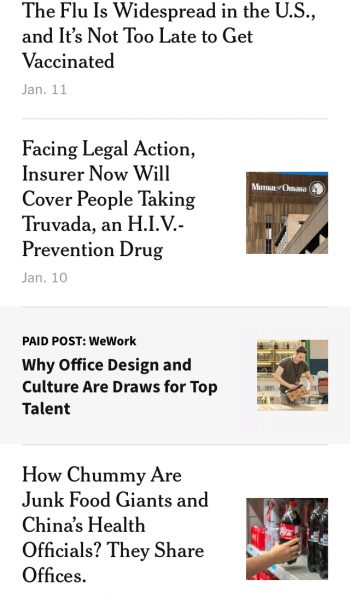An image resembling a clickable smartphone interface displays several articles in a tall, rectangular format. At the top, a bold headline reads, "The flu is widespread in the US, and it's not too late to get vaccinated," dated January 11th. Beneath a faint gray separator line, another bold headline states, "Facing legal action, insurer now will cover people taking Truvada, an HIV prevention drug," dated January 10th. To the right of this subheading, a square, brown-toned image appears, featuring a landscape reminiscent of Montana or Omaha.

Further down, the interface shows a section that appears to be clicked, marked by a slightly darker gray background. This section also contains faint gray lines in the backdrop. It is labeled with the bold text "Paid Post: WeWork," followed by the subhead, "Why office design and culture are draws for top talent." Another faint gray line separates this from the next headline, "How chummy are junk food giants and China's health officials? They share offices." Both of these latter articles come with accompanying images: one depicting a person holding a can of Coke, and the other showing a man pouring a beverage.